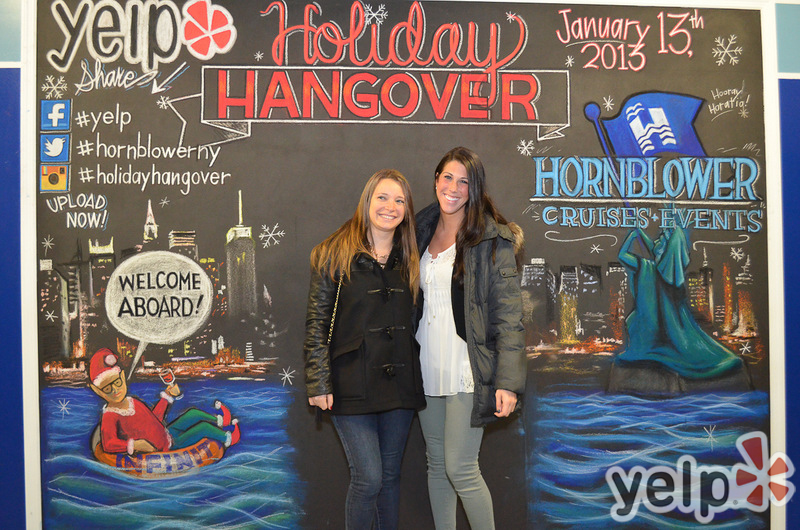In this vibrant, rectangular photograph taken outdoors during daylight, we see two women of Caucasian descent standing and hugging in front of a large, intricately designed banner. The woman on the left, shorter and possibly in her teenage years, boasts long, light brown hair parted at the side. She is dressed warmly in a black winter coat and blue jeans, radiating a youthful charm with her bright smile. To her right stands a slightly taller woman, perhaps in her thirties, with straight, dark brown hair. She is also smiling warmly, dressed in a gray winter coat that is open to reveal a white blouse, paired with light blue leggings. Both women exude joy and warmth against the festive backdrop.

The elaborate banner behind them is packed with colorful and detailed illustrations, depicting a whimsical holiday scene featuring a cityscape, an ocean, and a party atmosphere. At the top of the banner, "Holiday Hangover" is prominently displayed in bold red text with a white and black outline. In the upper right corner, the date "January 13th, 2023" is visible, alongside an image of the Statue of Liberty holding a blue flag with a white "H" and the words "Hornblower Cruises & Events."

On the left side of the banner, the Yelp logo and the word "Share" accompany the Facebook, Twitter, and Instagram logos, along with hashtags such as #Yelp, #HornblowerNewYork, and #HolidayHangover, encouraging viewers to upload their photos. An elf in a Santa costume is seen on an inflatable tube labeled "Infinity" with a speech bubble saying, "Welcome aboard." The overall atmosphere suggests a joyful, post-holiday celebration, perfectly captured by the smiles and the ambient energy of the two women in the image.